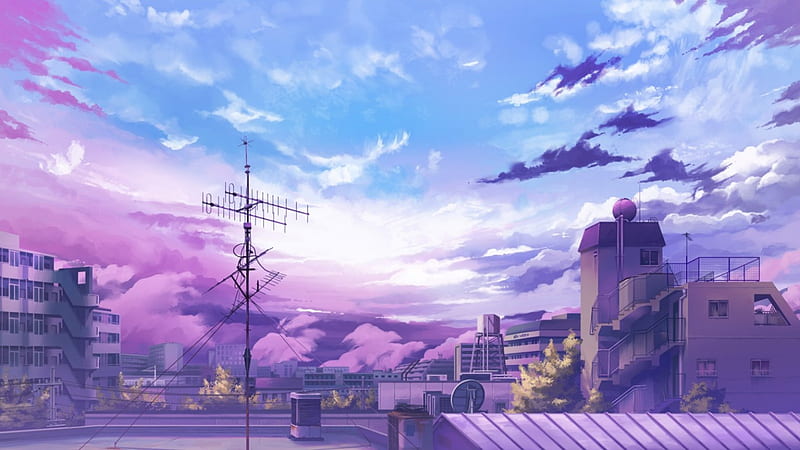This stylized, AI-generated rectangular painting showcases a rooftop view of a cityscape predominantly in hues of blue, white, and various shades of purple, with green accents of vegetation, including trees, towards the bottom of the image. The focus is on a vast sky filled with stark, high-contrast clouds, ranging from wispy to puffy formations. The perspective is from a rooftop, partially visible at the bottom of the frame, adding depth to the scene. Prominently featured in the left portion of the image is an ornate metal structure—likely an antenna—with wires extending into the sky. Below, the scene is populated by an array of brick and concrete buildings, including distinctive exterior stairscapes and what appears to be a large apartment building. The overall style is realistic but stops short of photorealism, encapsulating the serene yet dynamic essence of a city under a strikingly vibrant sky.